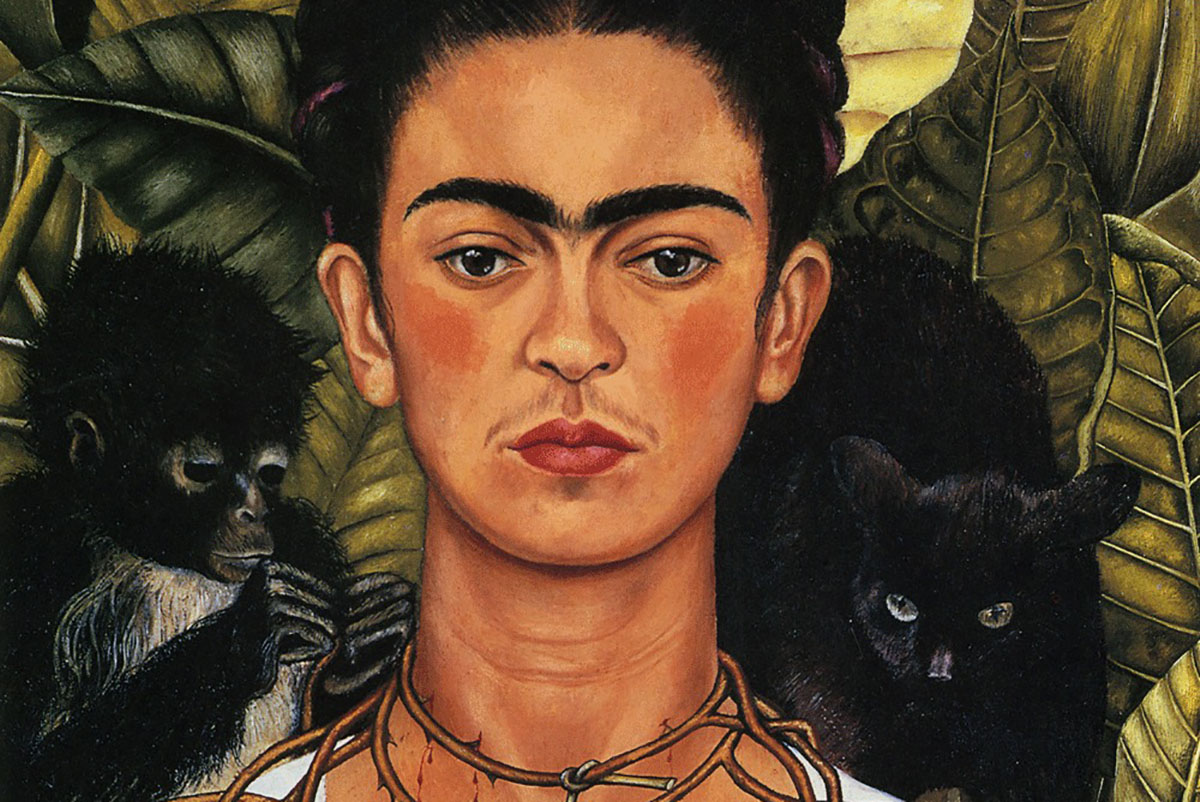The image is a detailed close-up portrait of a person, possibly the renowned Mexican artist Frida Kahlo, although the gender is somewhat ambiguous due to rounded facial features and minimal chin definition. The person has an expressive face with a serious, almost blank expression, and their hair is styled in a bun. They exhibit distinctive facial traits, such as thick eyebrows that meet at the center, a subtle mustache, a unibrow, rosy cheeks, and a hint of a mustache.

On their left shoulder rests a small black monkey with white fur on its front, suggesting it might be a baby monkey. On the right shoulder sits a mature black cat with heterochromia; one eye is a silvery color while the other is gold, and its nose has a purplish hue. Surrounding the individual are vibrant, dense jungle-like plants with dark green, brown, and yellow leaves, creating a lush, verdant backdrop. The entire image is brightly lit, clear, and richly colored, emphasizing the vivid details and textures of both the person and the surrounding foliage.